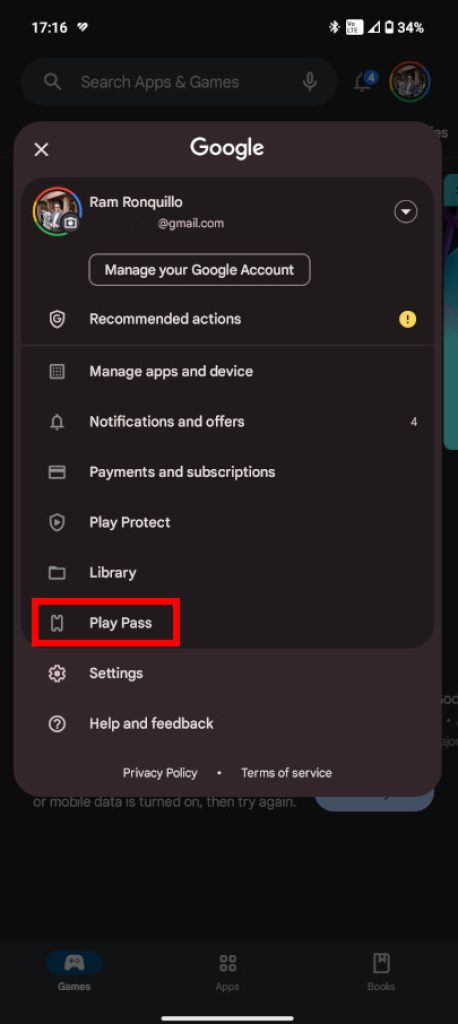The image appears to be a screenshot of a mobile device's settings or account management page, displayed in a dark theme with a black background and predominantly white text. 

At the very top left, the time is shown as 7:16, accompanied by a heart icon. On the top right, there are icons indicating Bluetooth status, mobile signal strength, and a battery level at 34%. Below this line, there is a greyed-out search bar reading "search apps and games," alongside an icon indicating four notifications. 

To the right of the search bar, there is a circular avatar with colored edges, possibly depicting a person in a blue jacket. 

A pop-up box with rounded edges features prominently at the center, with a greyed-out "X" at the upper left corner and the Google logo in the center. Beneath the Google logo, the same circular avatar reappears, revealing more details: the person wears glasses, possibly male, and appears to be dressed in a jacket. The associated email address is partially shown as "ronronico@gmail.com," with the first part blanked out. To the right of the email is a down arrow, followed by the option to "Manage your Google Account."

Below these details, a list of management options, each with small icons, is displayed:
1. **Recommended actions** with a yellow circle and black exclamation mark.
2. **Manage apps and device**
3. **Notifications and offers**
4. **Payments and subscriptions**
5. **Play Protect**
6. **Library**
7. **Play Pass**

Additionally, there is a red rectangle outlining this pop-up frame. Further navigation options include "Settings," "Help and feedback," "Privacy policy," and "Terms of service."

Towards the bottom, newer text mentions "on mobile data is turned on then try again," partially cut off by a blue button, indicating an error or notification message. At the very bottom of the screen, there are greyed-out navigation buttons for "Games," "Apps," and "Books," separated by a thin white line spanning one third of the screen's width.